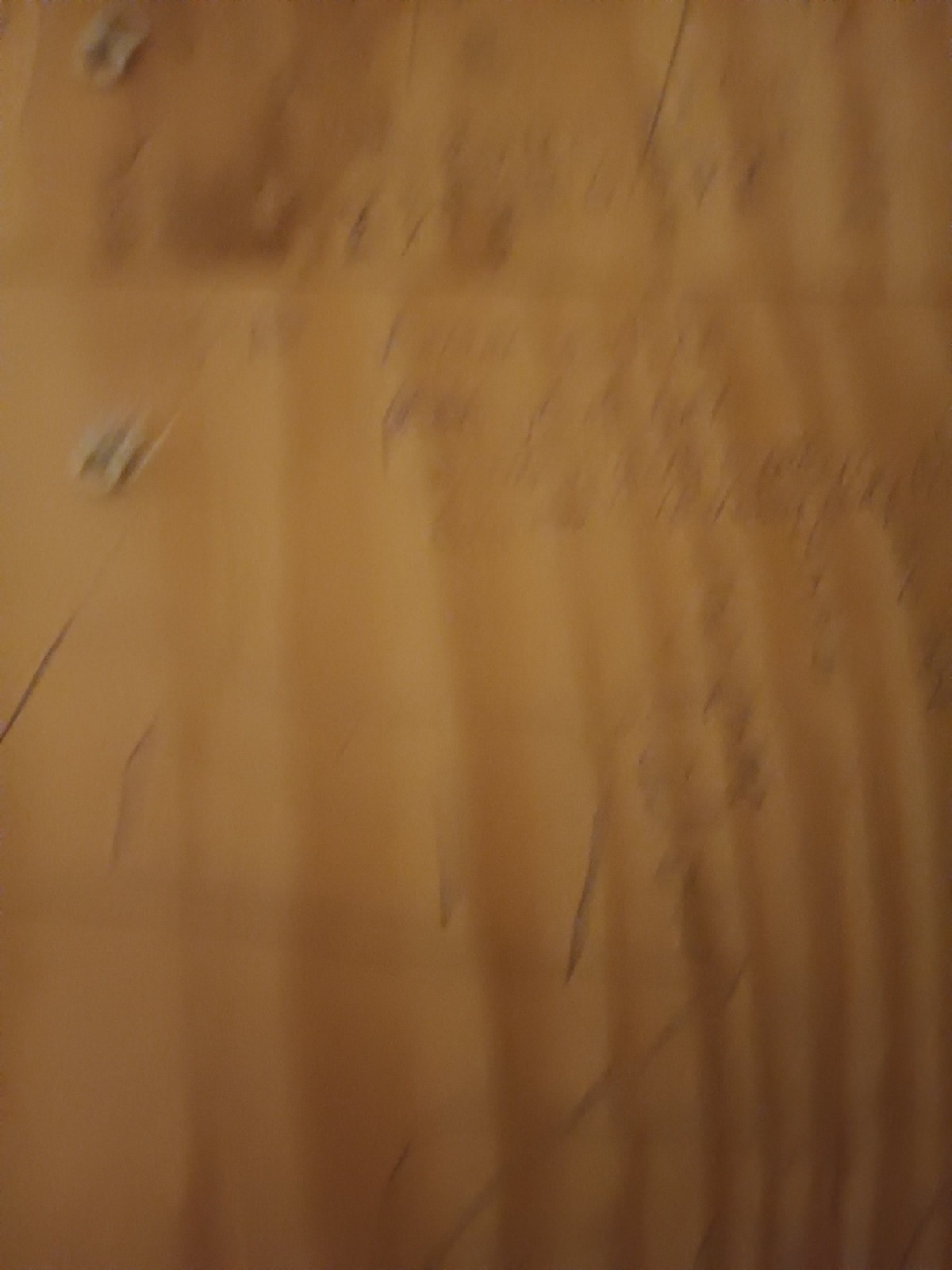This very blurry image predominantly features a light brown background that evokes the appearance of either old parchment or a dirt wall. The texture is marked by vertical lines or streaks that resemble wave patterns in sand, potentially caused by rippling effects. Scattered across the image are various faded markings and spots, including a noticeable number four and potentially other indeterminate letters or symbols. Indentations resembling scratches or scrapes are faintly visible. Two standout darker spots are located in the upper left corner, paired with random mottled brown coloration that lacks sharp, defining edges. The visual noise, such as horizontal streaks that resemble hairs, further obscures the overall clarity, giving the entire image a wrinkled or pleated look.